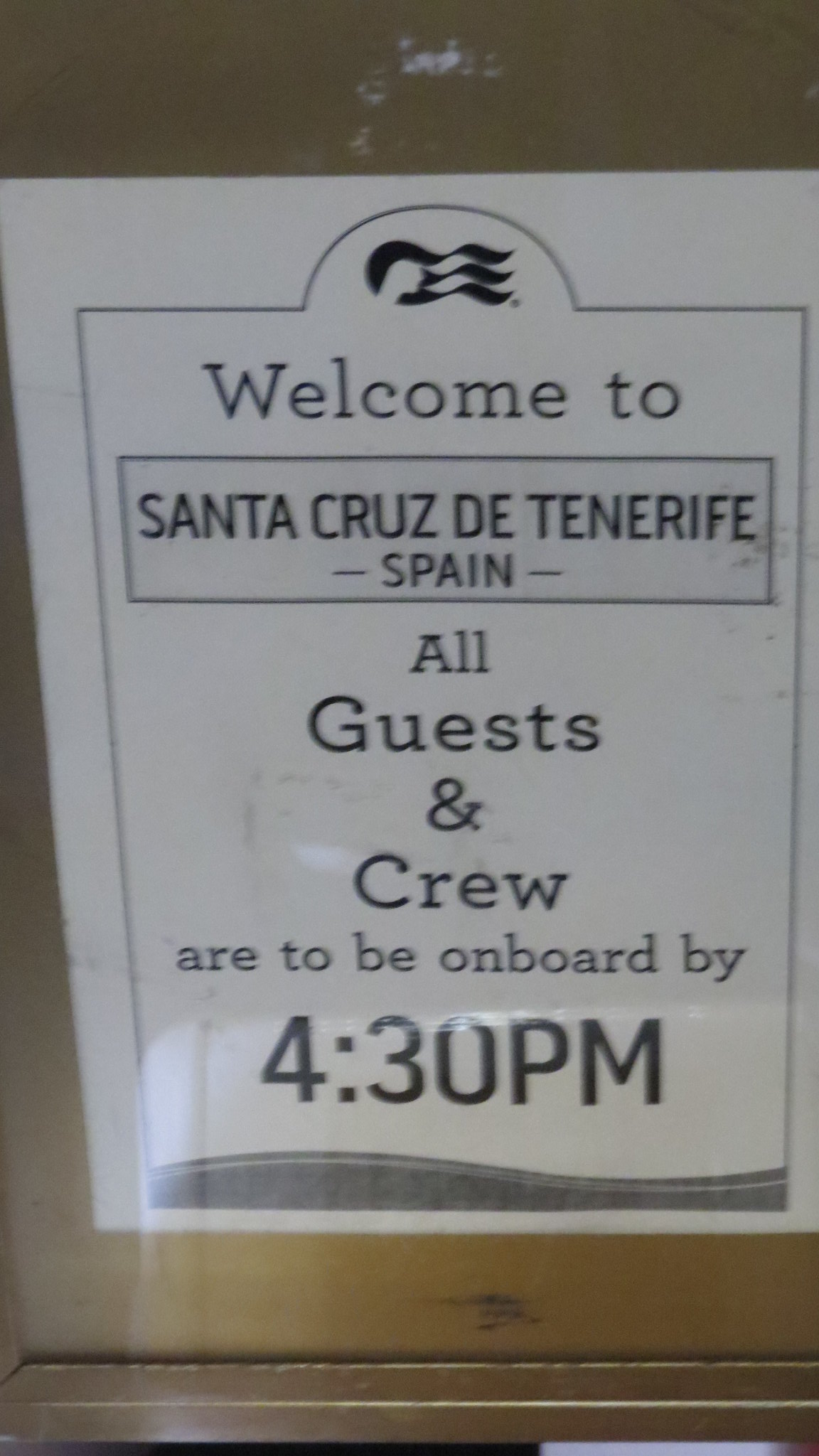The image depicts a black-and-white printed sign taped to a tan-colored wall or signboard. The sign reads, "Welcome to Santa Cruz de Tenerife, Spain. All guests and crew are to be on board by 4:30 PM." The plain, typefaced text is bordered and centered on the white paper, which features a logo at the top. The logo, appearing to represent a cruise ship company—possibly Princess Cruise Line—displays a woman's head with flowing waves. The tan background of the wall or signboard seems wooden and has a slightly golden, greenish-brown hue, adding a subtle contrast to the monochromatic sign.